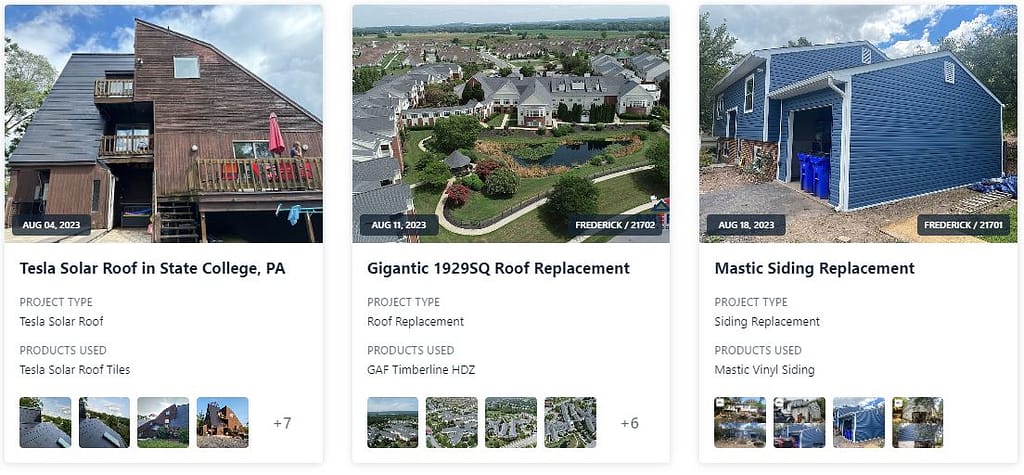The image is a collage of three project showcases, each detailed with descriptive captions and miniature images underneath.

On the left-hand side, there is a prominently featured image labeled "Tesla Solar Roof in State College, PA," with the project type specified as "Tesla Solar Roof." The products used for this project are "Tesla Solar Roof tiles." Accompanying this main image are four miniature photos, with a note indicating that there are a total of seven photos available for viewing. This project is dated August 4, 2023.

In the middle of the collage, another large image showcases a "Gigantic 1929 SQ Roof Replacement." The project type for this one is a "Roof Replacement," utilizing "GAF Timberline HDZ" products. Similar to the first project, there are four miniature images displayed beneath the main picture, accompanied by a notation that more images are available (a total of six additional photos). This project is dated August 11, 2023.

The third and final feature, on the right-hand side, displays an image with the heading "Mastic Siding Replacement." This project is classified as a "Siding Replacement," using "Mastic Vinyl Siding." Beneath this image, four miniature pictures are displayed, with no additional photos noted—indicating these are the only ones available. This project is dated August 18, 2023.